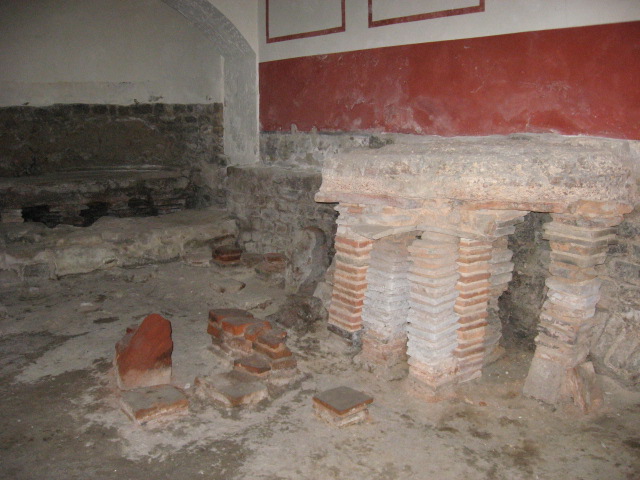The image captures an indoor setting of an old, ruinous room with a photographic style. The floor, predominantly gray and covered in splotches and dust, features stone elements with raised squares in the foreground. Positioned in the midground, there are several piles of stacked stone rectangles that form five columns, seemingly supporting a partially broken table. The table itself exhibits red and gray hues. The background reveals a white wall interspersed with two red rectangles and a red horizontal bar. In the top-left section of the image, a set of pews or a bench is visible beneath a white arch, hinting at a space that might once have been significant. The overall scene suggests a mixture of archaeological remnants and potential construction or demolition activity, with a focus on the aged and damaged concrete and stone structures scattered throughout. The image exudes a sense of historical decay, inviting speculation on its past and present state.